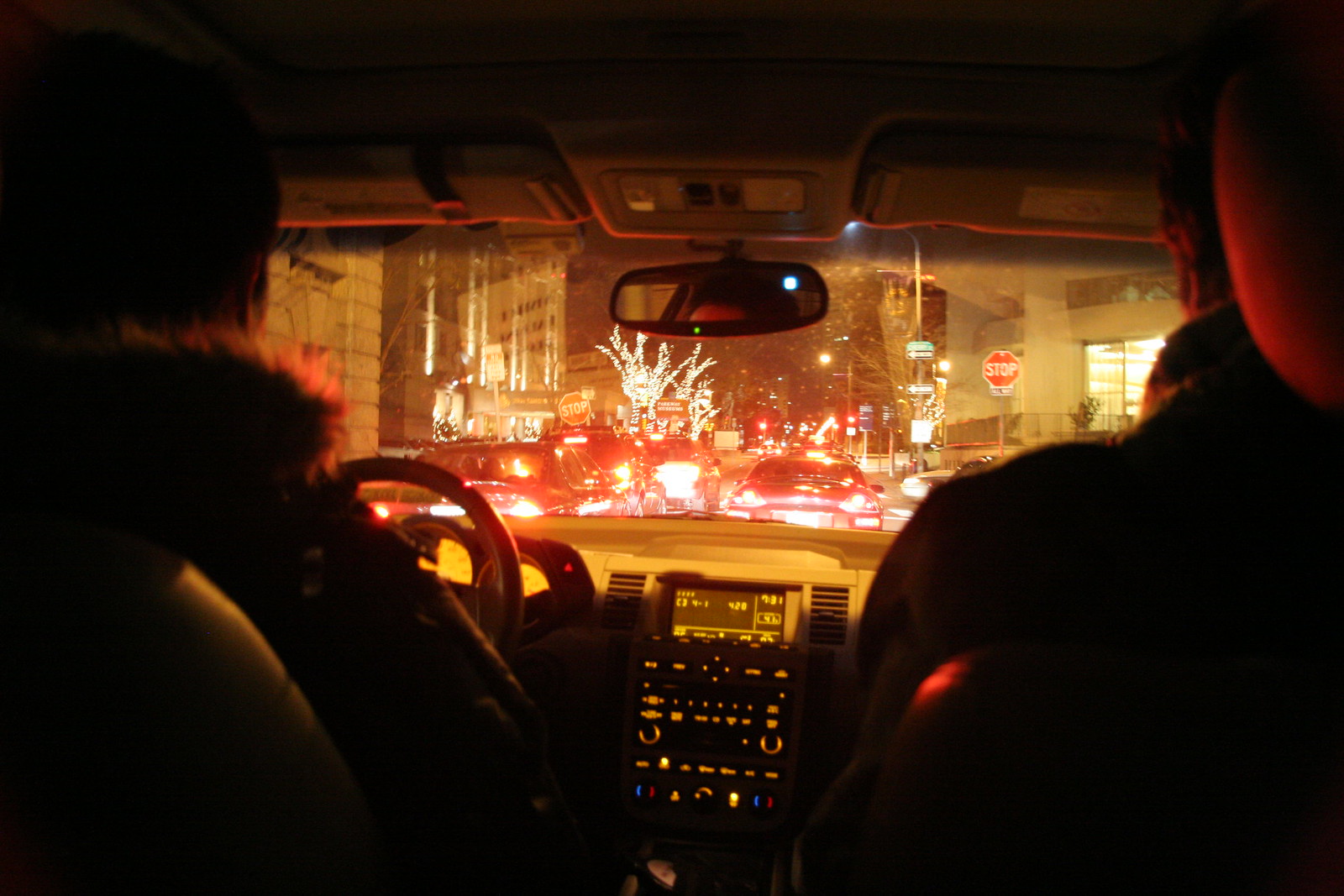The image captures an intimate moment inside a car, seemingly taken from the back seat. In the front, the driver is partially visible; they are wearing a coat with a furry hood and have short black hair. The silhouette of the driver is clearly outlined against the dim interior light. Next to the driver, the person in the passenger seat is leaning their head against the seat's headrest, also clad in a coat, and they appear to have short hair.

The dashboard and central controls of the car can be seen, along with the steering wheel. The vehicle's interior is modestly illuminated by the ambient glow of the street lights and festive decorations visible through the windows. To the right, the side mirror and a portion of the car’s roof with its visors closed can be seen. The scene outside the front windshield is filled with the vibrant essence of Christmas time; buildings adorned with festive lights, street lights twinkling, and a cascade of colors from car headlights and taillights fill the view. A stop sign is noticeable among the light display. The outer world contrasts starkly with the subdued silhouettes inside the car, casting a warm, celebratory ambiance overall.